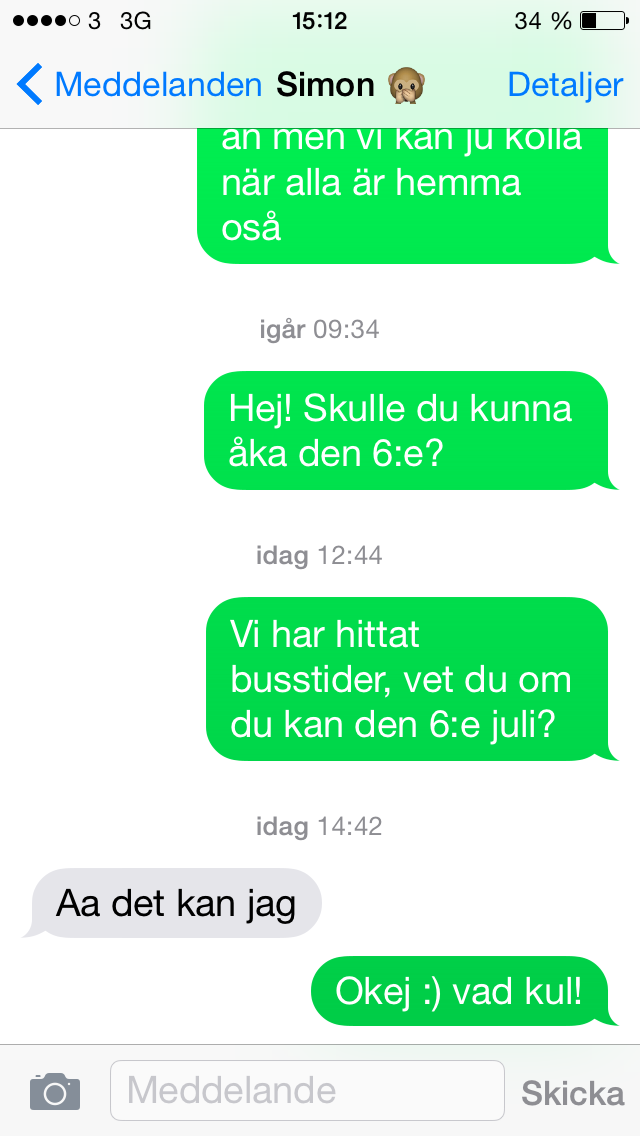This image is a detailed screenshot of a text message conversation in a foreign language, likely Swedish, taken from a smartphone. The screenshot captures a chat between two people, with the messages displayed in colorful speech bubbles against a white background. The outgoing messages are in bright kelly green bubbles with white text, while the responses are in gray bubbles with black text.

At the top of the screen, several status indicators are visible, including a 3G signal strength, the current time shown as 15:12, and a battery level at 34%. The header also includes the name "Simon" accompanied by a monkey face emoji, the word "Medellin," and another term "Detailjar," which seems to refer to the conversation's details.

The conversation consists of different time-stamped messages. One message from "Simon" reads "Igår 09:34 hej Sjula, du kanna, du kunna, uka den," and another response, time-stamped "Idag 12:44," reads "vi har hittat, boste der, vet du om du kan den, six, July." Lastly, there's a concluding reply marked by enthusiasm with a smiley face, "OK, OK, EJ, vad cool."

At the bottom of the screenshot, there is a text input area with a camera icon to the left and the words "Medelande" (likely intending "Meddelande," Swedish for message) along with "Skicka" (meaning send). The overall layout and visual indicators suggest a typical smartphone interface for text messaging.